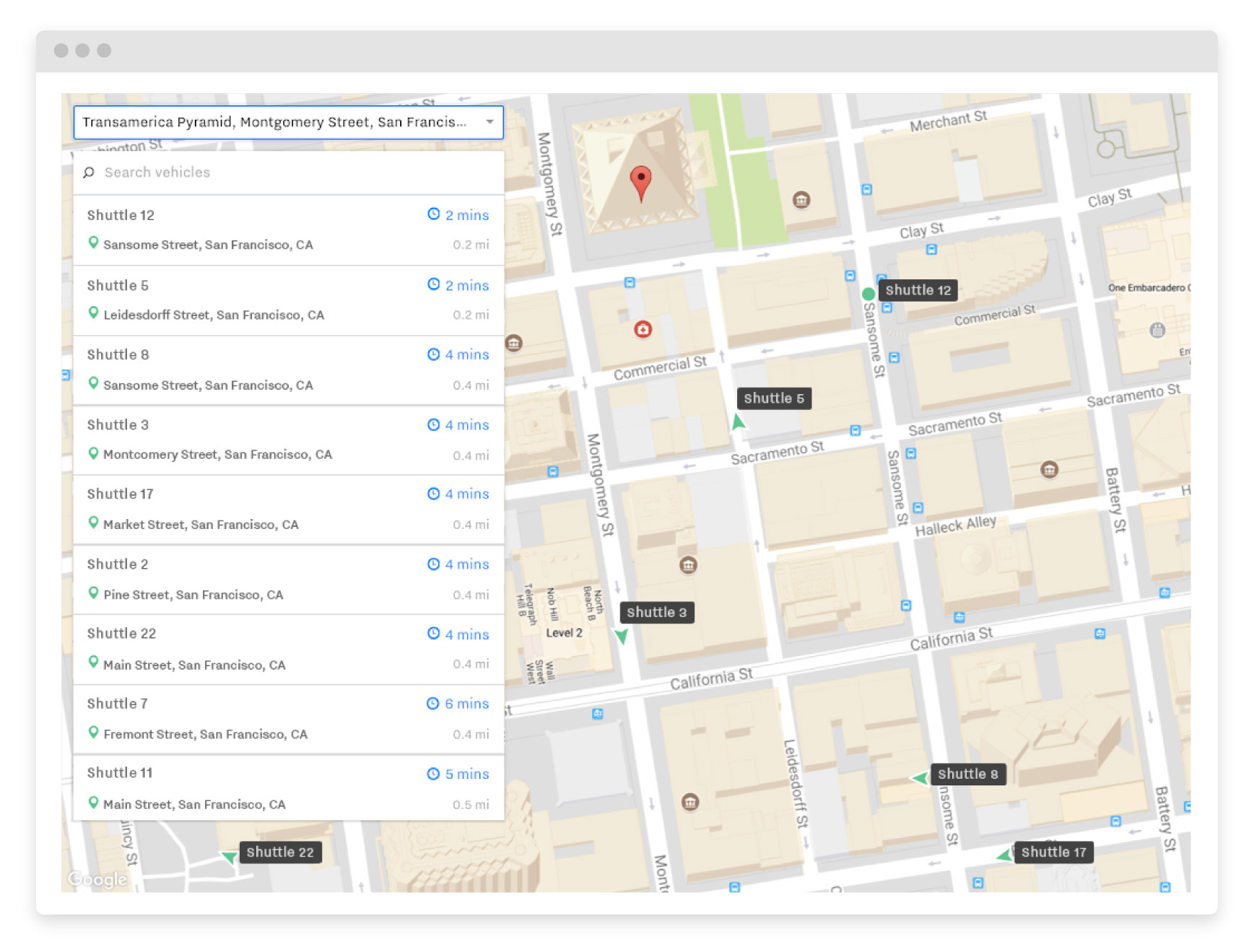The image displayed is an aerial view of a GPS-like map showcasing the street layout. A prominent grey bar extends horizontally across the upper part of the map, from left to right. Overlaying the left-hand side of the map is a search bar featuring a drop-down arrow, with the text "Transamerica Pyramid, Montgomery Street, San Francisco" displayed within it.

Below this search bar, there is another text field labeled "Search Vehicles." This section lists nine selectable options vertically aligned, each corresponding to a shuttle with specific details. The first entry is "Shuttle 12," indicating its arrival in 2 minutes and its distance of 0.2 miles. Subsequent entries list various other shuttles: "Shuttle 5," "Shuttle 8," "Shuttle 3," "Shuttle 17," "Shuttle 2," "Shuttle 22," "Shuttle 7," and "Shuttle 11." Each shuttle is clearly labeled for easy identification.